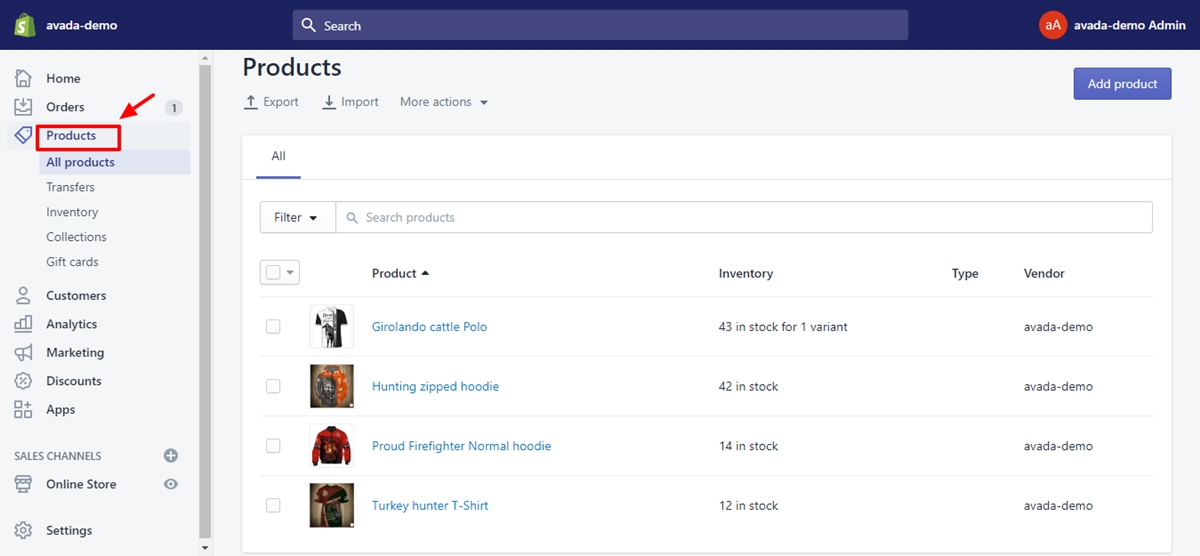**Caption:**

This image is a detailed screenshot of an admin dashboard labeled "Avada Demo." In the upper left-hand corner is a blue rectangle featuring a green shopping bag icon with an S or dollar sign, next to the text "Avada Demo." Alongside it, on the right, is a search bar in a lighter blue and a red circle with white lowercase and capitalized "A" letters. Adjacent to these elements, "Avada Demo Admin" is displayed.

On the left side, a comprehensive vertical menu lists multiple options: Home, Orders, Products (highlighted with a red square and arrow), All Products, Transfers, Inventory, Collections, Gift Cards, Customers, Analytics, Marketing, Discounts, Apps, Sales Channels, Online Store, and Settings.

In the main content area to the right, the page title "Products" sits at the top. Next to it are an up arrow labeled "Export," a down arrow labeled "Import," and a "More Actions" button with a dropdown arrow. Below this, a blue rectangular "Add Product" button appears.

Further down, the interface shows filtering options and a search bar beneath the "All" tab, indicated by a bluish underline. Below this, a table displays product details in columns labeled "Products," "Inventory," and "Vendor." Listed items include a "Girolando Cattle Polo Hunting Zipped Hoodie" with 43 in stock, "Proud Firefighter Normal Hoodie" with 42 in stock, "Turkey Hunter T-shirt" with 14 in stock, and another item with 12 in stock. The "Type" column is empty, while the "Vendor" column lists all items under "Avada Demo."